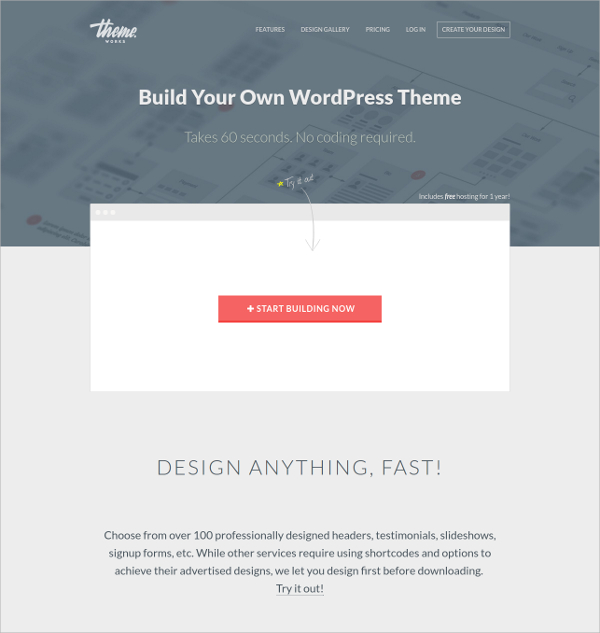The image depicts a website interface. In the top left corner, the word "Theme" is visible with an unreadable, blurred word beneath it. The navigation bar at the top includes menu items "Features," "Design Gallery," "Pricing," and "Login," all in white font against the darker background. Additionally, there's a prominent box with the text "Create Your Own" also in white font.

The upper half of the webpage features a blurred image background that appears to display either truth tables or flowcharts of various forms. Centrally positioned over this image is a bold, white headline stating "Build Your Own WordPress Theme." Directly beneath this, in a slightly lighter font, is the subheading "Take 60 seconds, no coding required."

At the center of this section, there is a prominent white box containing a bright red button with a plus sign, labeled "Start Building Now" and an adjacent arrow with the text "Try it out."

The bottom half of the webpage transitions to a gray background. It features the phrase "Design Anything Fast" in black font. At the base of this section, promotional text reads "Choose from over 100 professionally designed headers, testimonials, slideshows, signup forms, etc. While other services require using shortcodes and options to achieve their advertised design, we let you try out first before downloading." This section also includes a button labeled "Try it out."